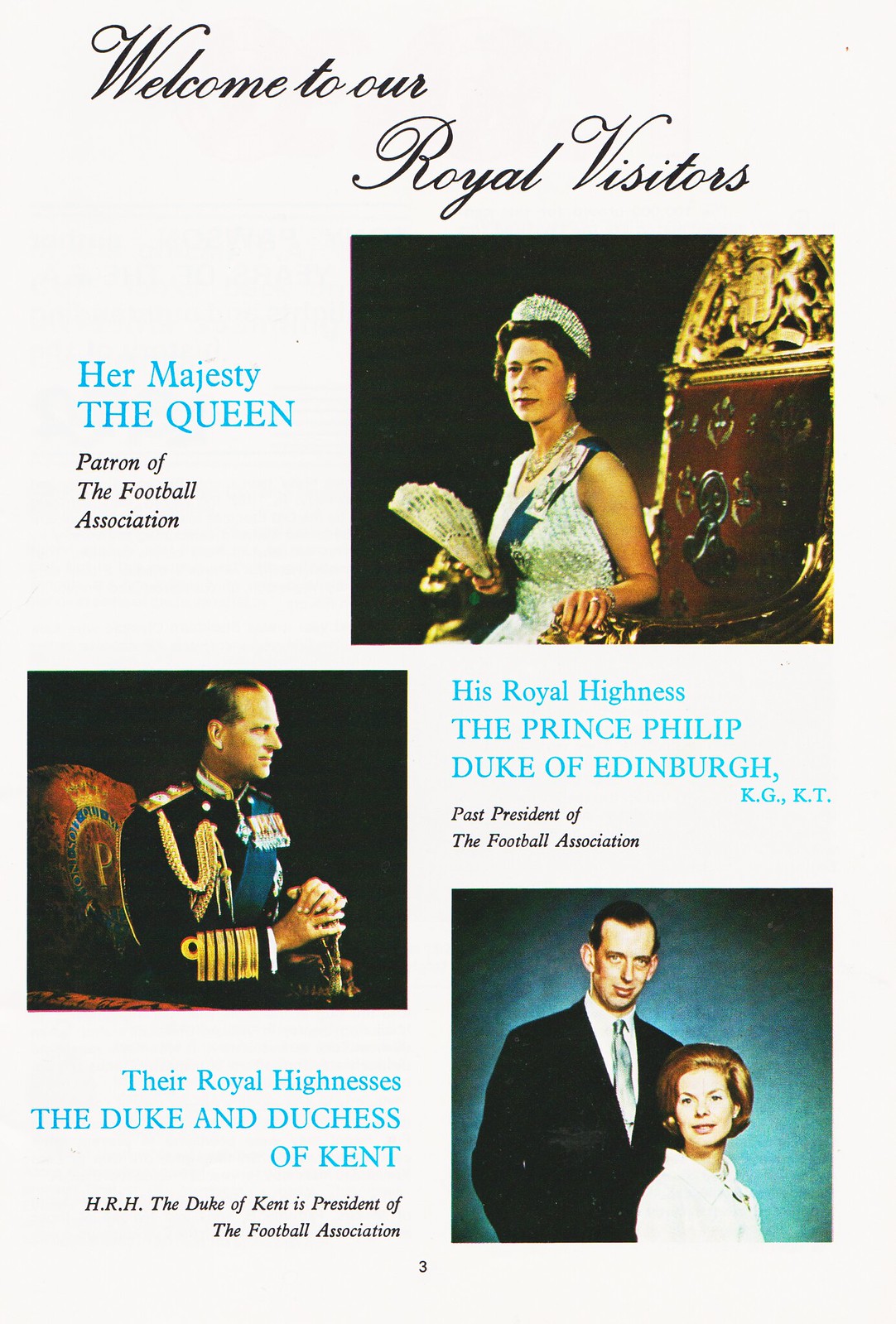The flyer, printed on light gray paper in portrait mode, warmly welcomes its readers with the cursive text "Welcome to Our Royal Visitors" at the top. Beneath this heading, the flyer features three photographs of distinguished individuals, each accompanied by descriptive captions in light blue and black text. 

At the top center, there is a photograph of an older woman, who is presumably the Queen, adorned with a crown and holding a folding fan while seated on a red and gold throne. To her left, the caption in blue text reads, "Her Majesty the Queen," and below that in black text, "Patron of the Football Association."

In the middle of the flyer, there is a photograph of a man in a military uniform sitting on a matching red and gold chair. To his right, the blue caption reads, "His Royal Highness The Prince Philip, Duke of Edinburgh KGKT," followed by a black text caption, "Past President of the Football Association."

Below this, towards the bottom of the flyer, there is a photograph of the Duke and Duchess of Kent. The caption to their left states in blue text, "His Royal Highness, the Duke of Kent," and in black text, "President of the Football Association."

Accenting colors of light blue, red, gold, and black punctuate the minimalist backdrop, creating a distinguished yet welcoming presentation for this royal-themed event.